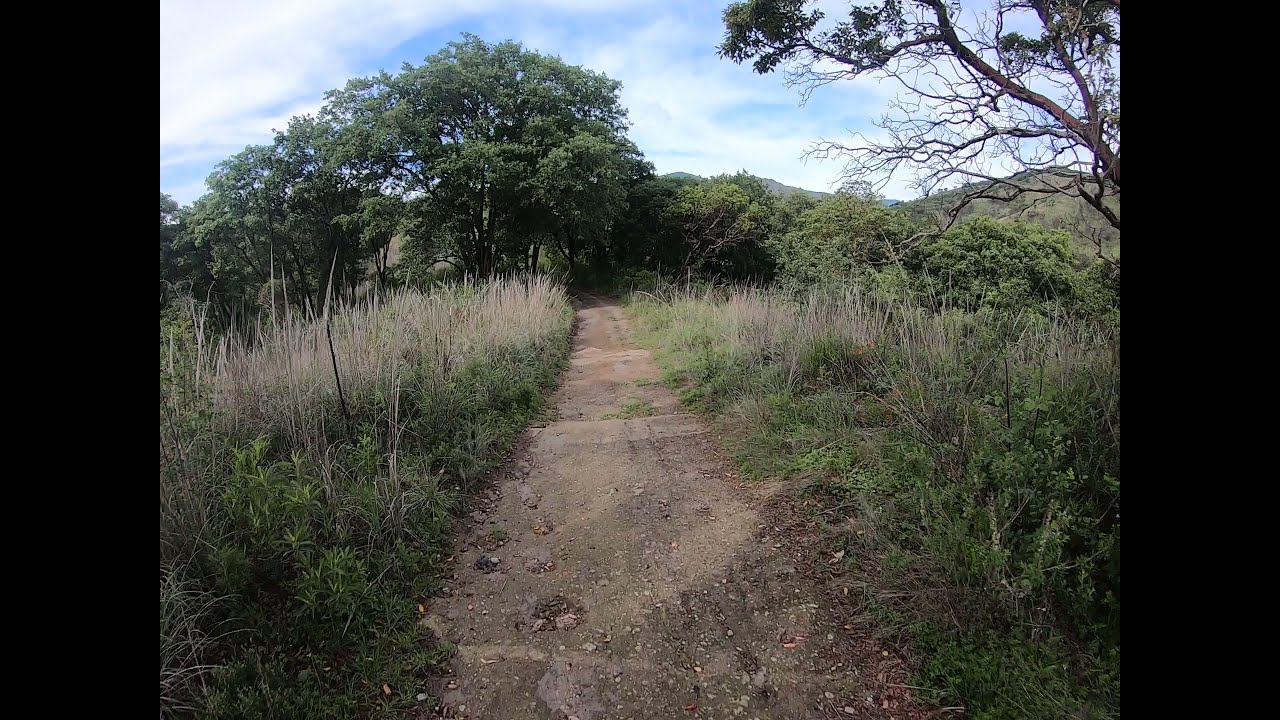The image depicts a dirt road cutting through dry, sparse vegetation with a backdrop of gently rolling hills blanketed in green. The sky above is a light blue expanse dotted with wispy white clouds, lending a serene atmosphere to the scene. The road itself is predominantly brown and rocky, interspersed with dark patches and flanked by brown, green, and tan grasses standing about two to three feet tall. The vegetation comprises thin trees with dark green leaves, and on the top right forefront, there’s a mostly bare tree branch with a few clusters of dark green leaves. The left side of the road is marked by piles of dry, crumbly mud-like substance and spiky weeds. Despite the greenery, there's a noticeable dryness to the surroundings, with some of the plant life appearing parched, reminiscent of semi-arid regions like the Sahara or parts of Africa. There's no sign of animals, humans, or any form of civilization, adding to the solitary beauty of the landscape.